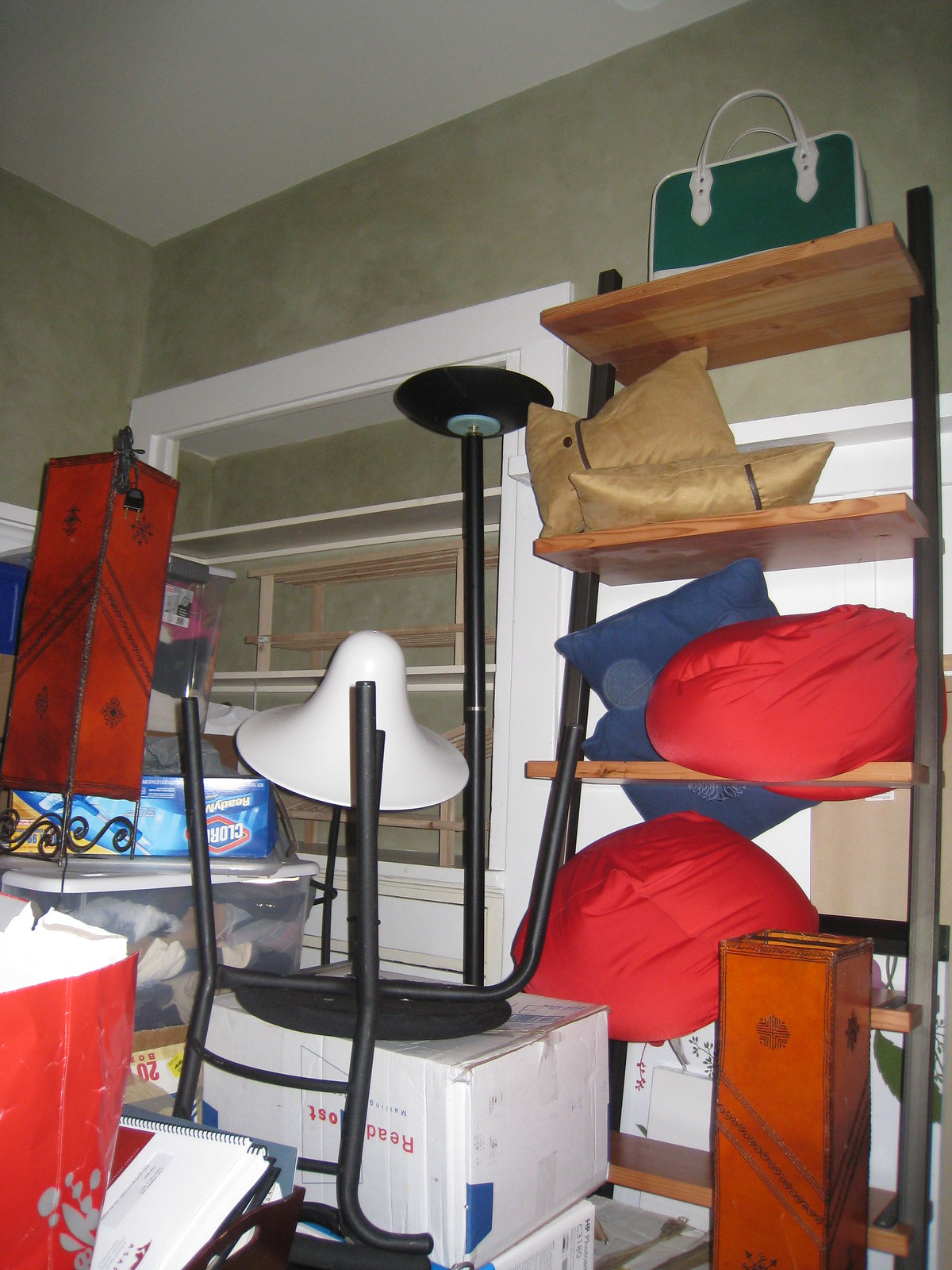The image depicts a cluttered storage area, possibly a room, a closet, or a garage, filled with various items. In the foreground, there's a wooden shelf supported by steel beams, holding four pillows—two blue and two gold. The shelf also contains two small red bean bags placed on different levels. At the top of the shelf, a green purse with white straps is visible next to a tall black lamp. There is a red object with a plug that resembles a light, although its exact purpose is unclear.

Additionally, a container of Clorox wipes, presumably meant for a mop, is visible among the items. Various boxes are scattered around, including two white boxes with blue and red lettering, stacked on top of each other. An upside-down chair is placed above these boxes. A red bag and another red lamp-like object can be seen, though the floor remains out of view. Clear plastic boxes are also stacked together, and another shelf, apparently empty, is part of the scene. The overall impression is one of disarray, typical of a storage space in need of organization.